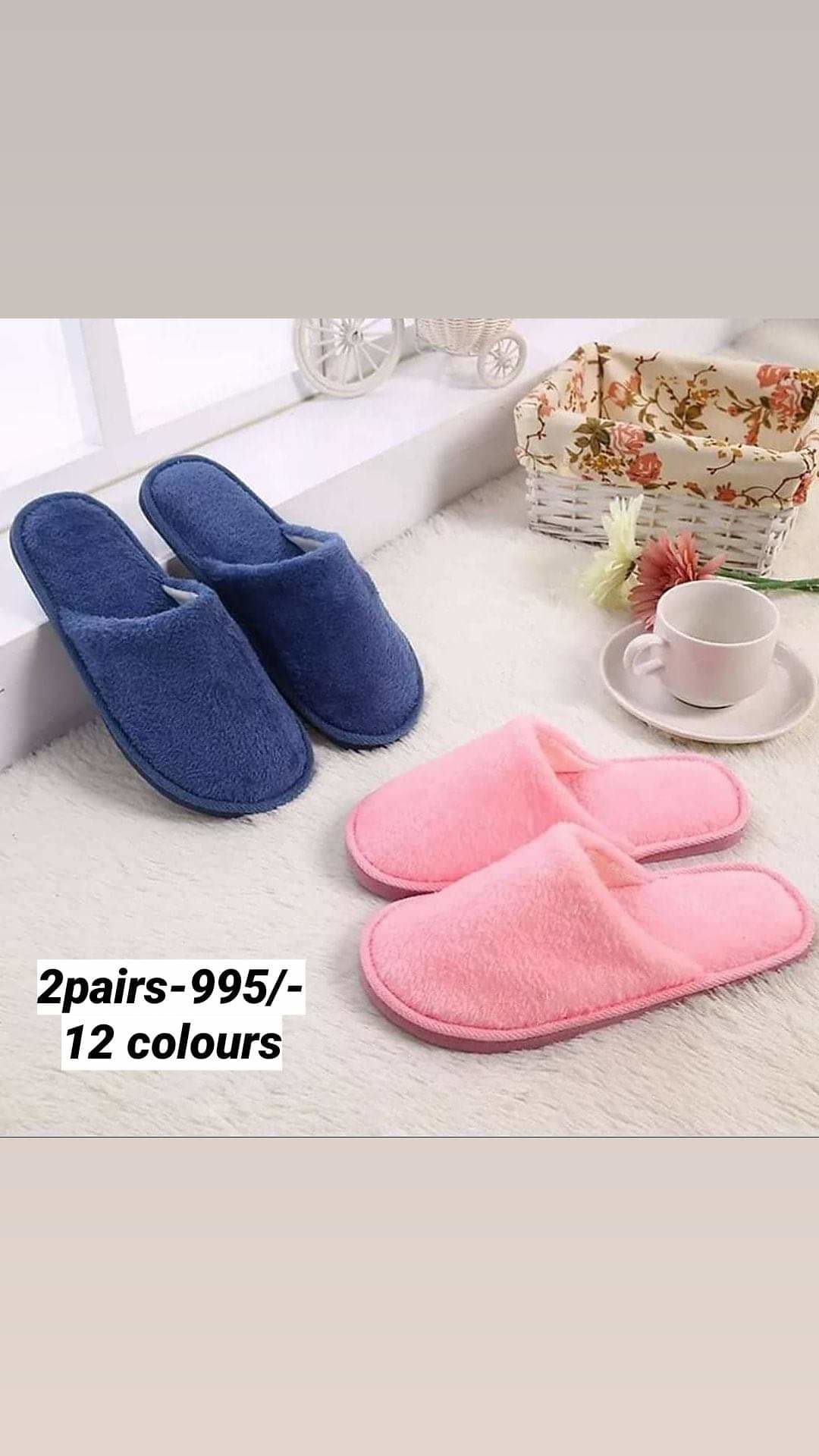This photograph, likely an Instagram short, features a cozy, indoor scene centered around fuzzy slippers. It appears as a square image with a gray void around it, giving the impression of a phone screenshot. The image showcases two pairs of fuzzy slippers positioned on a soft, white, rug-like carpet. A pair of navy blue slippers are upright, leaning against a white windowsill in the upper left corner. Below them, in the lower right corner, is a pair of pink slippers, designed to cover the toes while leaving the back open.

In the upper section of the image, above the pink slippers, a white, pattern-free ceramic teacup rests on a matching saucer, creating a homely feel. To the top right, a white wicker basket with a floral print cloth inside complements the scene. Text in black on a white background is visible in the lower left, reading "two pairs 995/12 colours," with the British spelling of "colors." The overall composition, along with the descriptive text, suggests that this is likely an advertisement for the slippers.